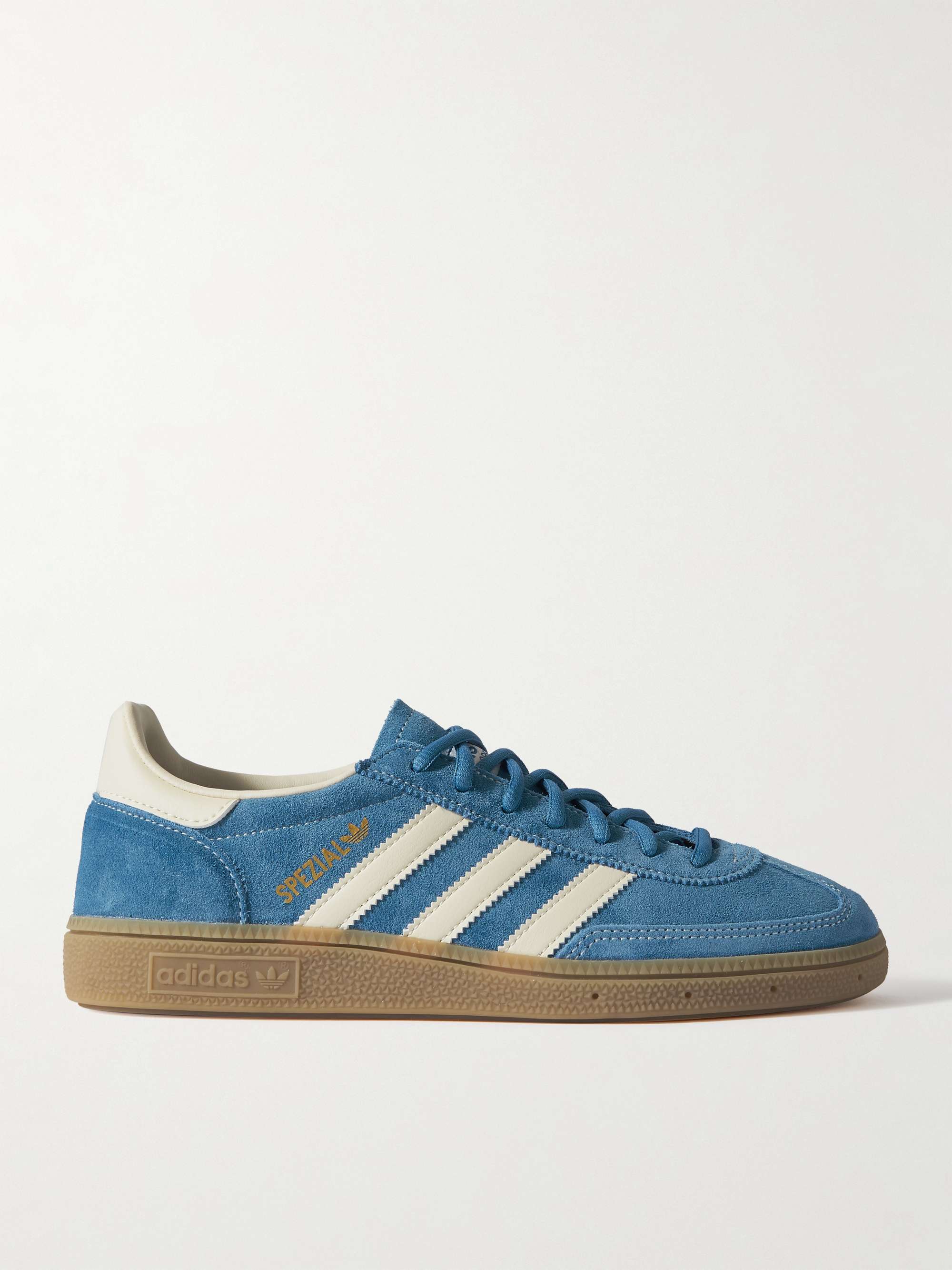The photo features a side view of a blue Adidas sneaker, prominently showcasing its detailed features on a gray background. The upper part of the shoe, which appears to have a velvety or suede texture, is blue and adorned with three iconic white stripes along the side. The laces, also blue but slightly darker than the shoe itself, contribute to its sleek design. The heel area and the top back part of the shoe are highlighted in white, complementing the stripes. The shoe rests on a thick, tan brown sole, which is branded with the Adidas logo. Additionally, the shoe bears the text "SPEZIAL" in light brown, hinting at a special edition or collection. The entire composition of the image emphasizes the distinctive and stylish elements of this Adidas sneaker.